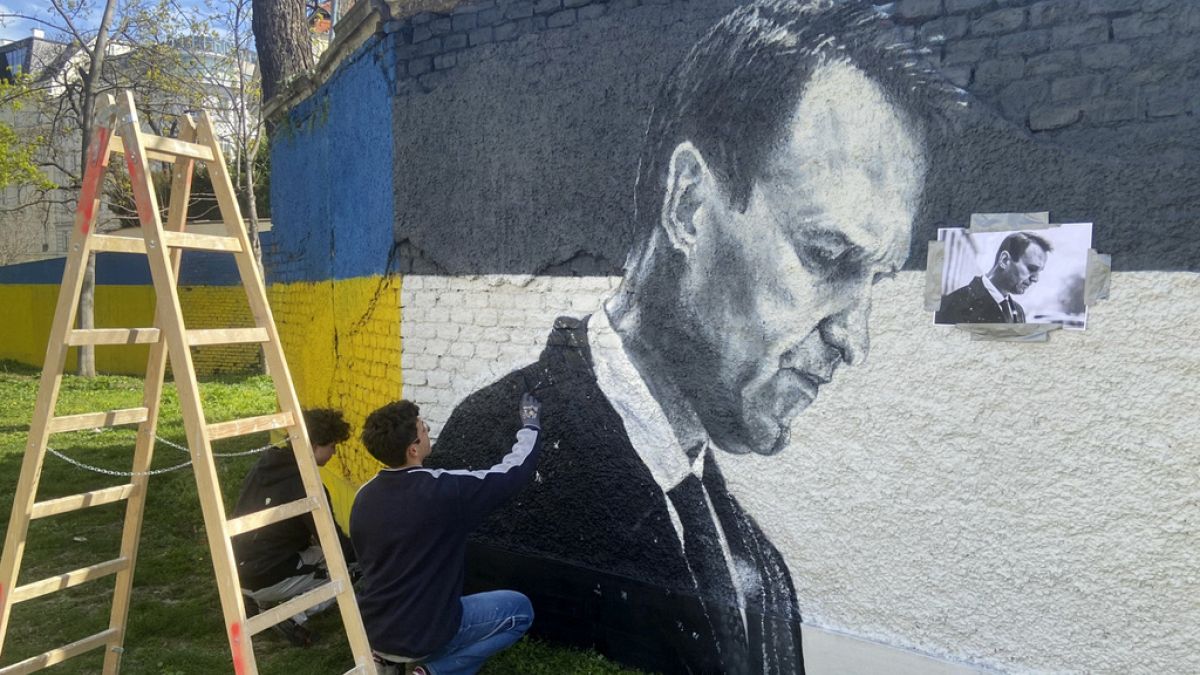In this detailed horizontal photograph of an outdoor mural project, two artists are captured in the midst of painting a large, partially colored brick wall. The mural prominently features a black and white portrait of an unidentified man in his 40s or 50s, characterized by his short-cropped hair, black suit with a white collar, and black tie. The man in the mural appears to be looking down, and a photograph of him, serving as a reference, is taped to the wall nearby.

The wall's background transitions from dark gray to light gray in the section featuring the mural, then shifts to a vibrant yellow and blue lower down. The artists, both with short hair, are working on their knees. The primary artist, wearing a black jacket and jeans, is focused on painting the man's jacket, while his assistant, dressed in a black top and either white or gray pants, is contributing to the yellow and blue sections of the wall. 

A light tan wooden stepladder stands behind the artists, and the scene is set against a backdrop of tall white concrete buildings, which are partially visible in the upper left corner of the image. The grassy area nearby basks in sunlight, and we can also see a yellow and blue fence extending across the yard. A few scattered trees with green leaves add a touch of nature to the urban environment.